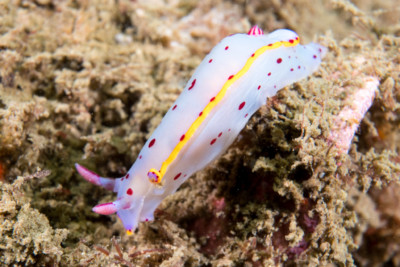The image depicts a close-up view of a uniquely colored white slug, featuring vibrant pink tentacles and distinctive red dots scattered across its body. A prominent yellow stripe runs down its back, adding to its striking appearance. The slug is moving to the left, crawling over a surface that appears to be dirt or sand, given its brownish-tan color and clumpy texture. There are no other discernible objects such as foliage, sky, or ground visible in the image, and the slug’s head is not clearly seen. The overall close-up nature of the photo highlights the slug’s slimy and mushy texture, which might make it reminiscent of underwater creatures, although it is primarily observed in a terrestrial context.